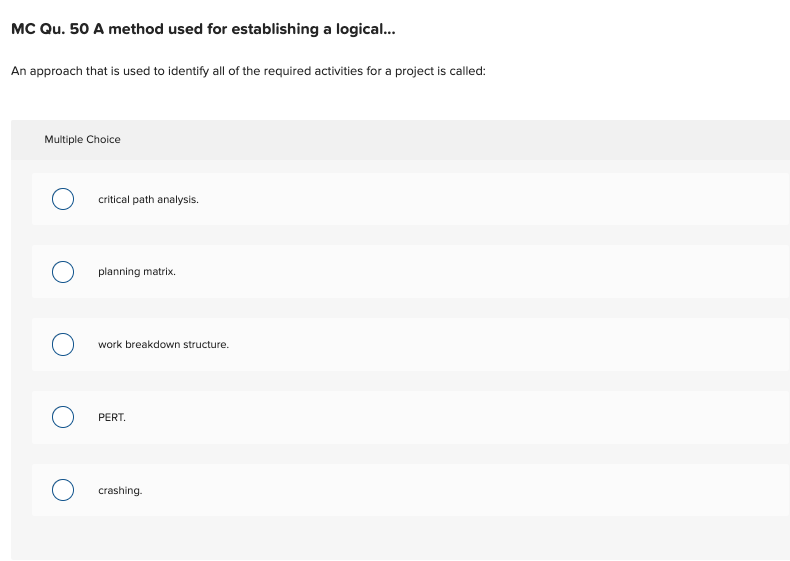This screenshot captures a segment of a standardized test question. Positioned in the top left corner, outside the main content, is the label "MCQU.50," indicating the type or number of the question. Below this label, in smaller text, is the partial description: "a method used for establishing a logical...” and beneath that, the full description: "an approach that is used to identify all of the required activities for a project is called:"

Directly below the question itself, a light gray box contains the multiple-choice options. Each option is encased in a slightly lighter gray box, presenting an alternating pattern for visual distinction. In the upper left corner of this choice box, "Multiple Choice" is written, with the letters "M" and "C" capitalized.

The answer choices listed are:
1. Critical path analysis.
2. Planning matrix.
3. Work breakdown structure.
4. PERT (in all caps).
5. Crashing.

Each choice is followed by a period. To the left of these options, there are empty circles intended for respondents to mark their selected answer.